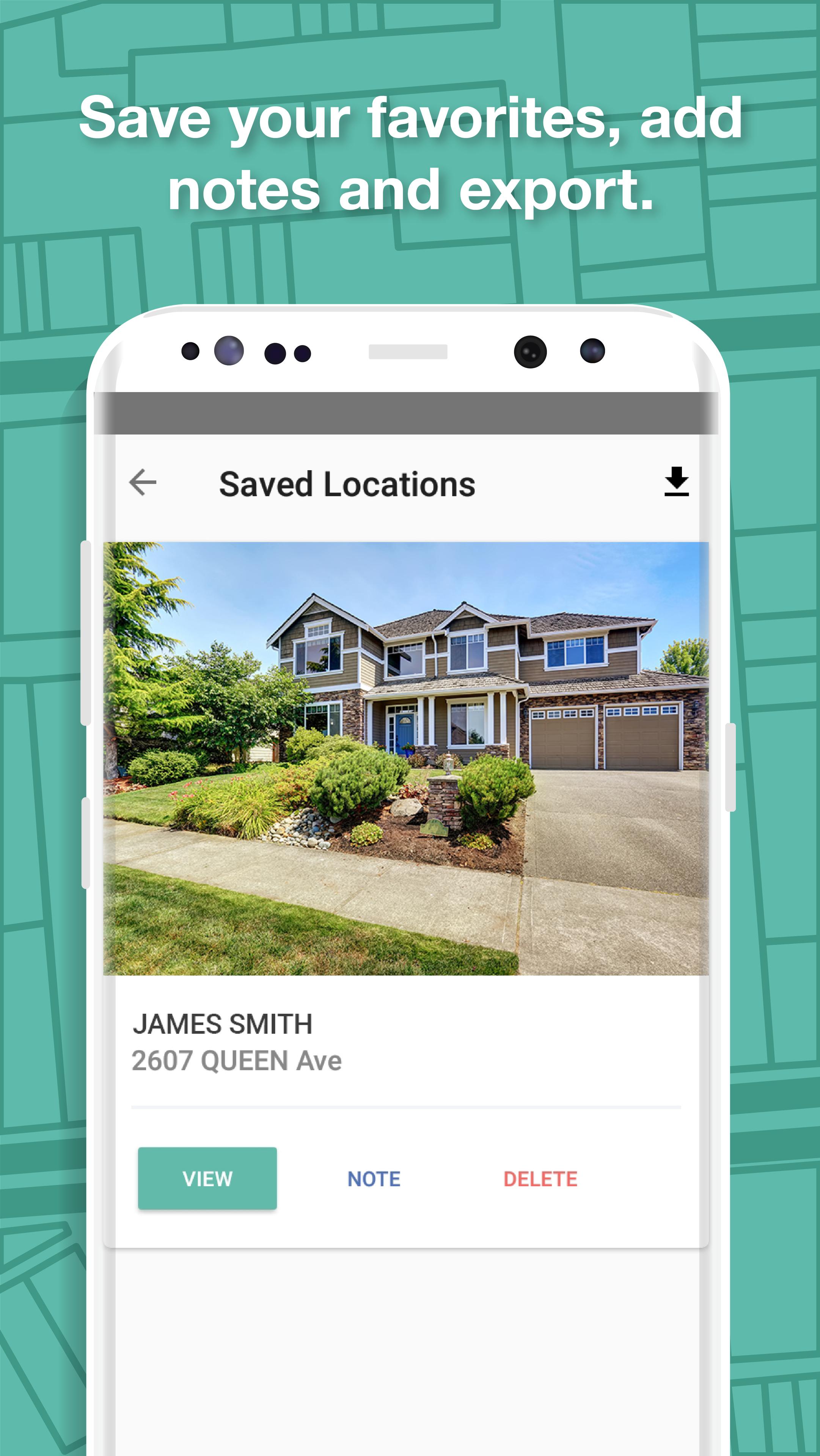The image features a teal-colored background adorned with various rectangular and square shapes of differing sizes, arranged haphazardly without any discernible pattern. At the top, written in white text, are the words: "Save your favorites, add notes, and export."

Below this text, there is an illustration of a smartphone screen. The top of the screen displays the phrase "Save Location," flanked by a left-pointing arrow on the left and a download button on the right. Beneath, the smartphone screen shows a photograph of a large, dark grayish-brown house with a two-car garage. The bottom floor of the house features a stone exterior, while the upper part appears to be tiled, although the image is small and the material is not entirely clear. The photograph also includes details of a driveway, some trees and bushes, a sidewalk, and a grassy area.

Underneath the house image, text reads "James Smith, 2607 Queen Avenue." Below this, there are three buttons matching the teal background color. The buttons are labeled "View," "Note" (in blue), and "Delete" (in red).